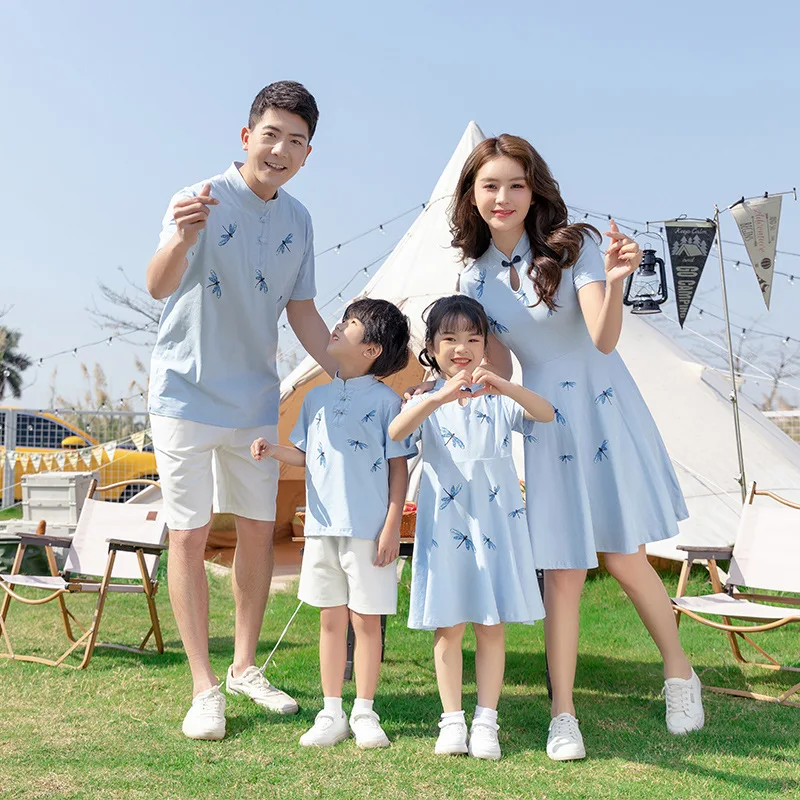The photograph captures a joyful moment of an Asian family of four standing on a lush green grassy field. The family is positioned with the father on the left, the son to his right, followed by the daughter, and the mother on the far right. The father has dark black hair, and the mother’s long hair falls past her shoulders down to her chest. All family members are wearing coordinated outfits featuring a light blue color adorned with royal blue dragonfly patterns. The males are dressed in light blue t-shirts paired with light cream shorts and white sneakers, while the mother and daughter wear matching light blue dresses with the same dragonfly design and white sneakers. 

In the background, several foldable wooden and canvas white chairs are visible. Behind the family, there is a white teepee decorated with string lights, pennants, and a lantern hanging. The boy gazes up at his father, while the daughter forms a heart shape with her hands, and the parents wave with one hand raised in a friendly gesture. The scene appears to be set at an outdoor festivity, evident from the decorative elements like the tents and banners strung around. Off to the right side, a yellow car is partially visible, adding to the cheerful and celebratory atmosphere of the photograph.